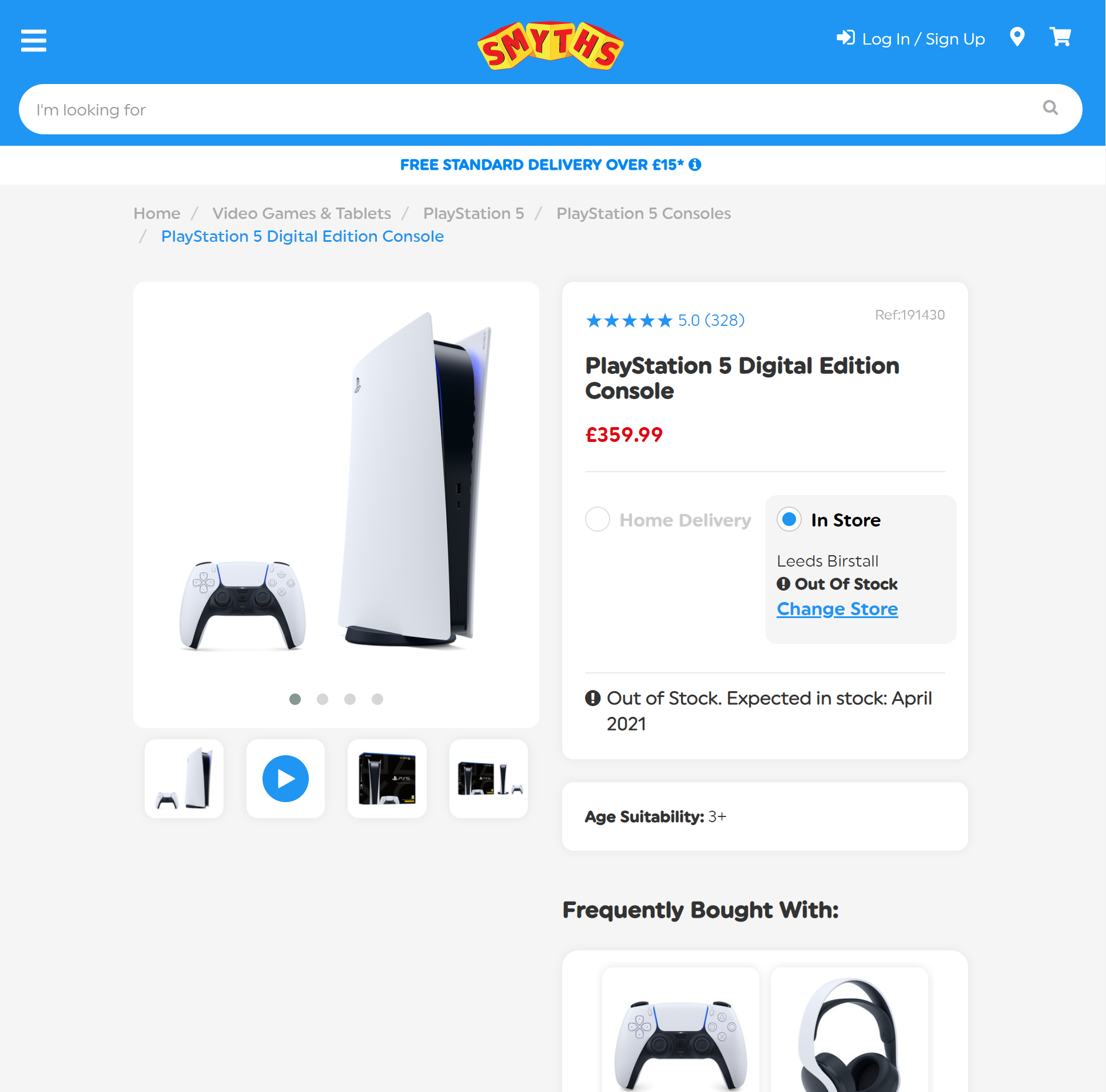The upper section of the image features a bold blue background adorned with three small horizontal lines on the left side. Centrally displayed, the word "SMYTHS" is prominently spelled out in yellow and red blocks, indicative of the Smiths brand. Beneath this heading, a long search bar extends across the design. Directly below, in matching bold blue text, is the message: "Free Standard Delivery over €15."

Dominating the center of the image is a vertical display of the PlayStation 5 console, characterized by its sleek white and black color scheme. To the left of the console, the matching white and black controller is visible. To the right of the console, five blue stars are shown, followed by the number (328) in parentheses, highlighting customer reviews.

Just below, bold black text reads "PlayStation 5 Digital Edition Console," and directly under this is the price, prominently displayed in red at €359.99. 

Further down, the caption indicates availability options starting with "Home Delivery." Adjacent to this is a blue circle, and beside that, it states "In Store," followed by "Leeds Burstall." Next to this is a black circle containing an exclamation point, with the text "Out of Stock" beside it. 

Toward the bottom, the text "Change Store" is underlined in blue, accompanied by the note "Out of Stock, Expected In Stock April 2021."